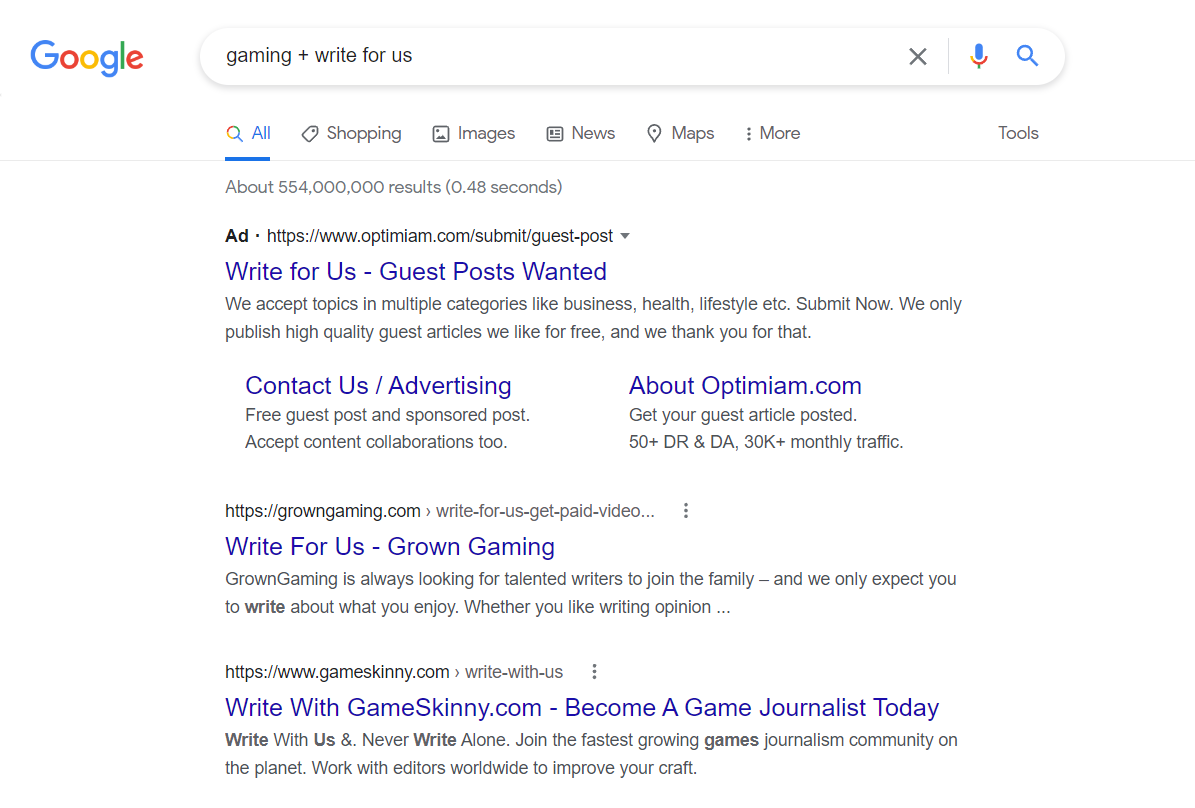The image depicts a Google search results page. In the top left corner, the recognizable Google logo is displayed. Beneath the logo, the search query "Gaming Plus Right for Us" is visible in the text bar. Directly below the search bar, the "All" search option is selected, with other options such as Shopping, Images, News, and Maps lined up beside it.

The first search result features a link titled "Right for Us," which invites guests to submit posts. The accompanying description highlights that the site accepts topics in various categories, including business, health, and lifestyle. It also emphasizes a commitment to publishing only high-quality guest articles for free, and it offers thanks to contributors. Additional links like "Contact Us," "Advertising," "Free Guest Posts and Sponsored Posts," and a note about accepting content collaborations are listed underneath. To the right, the text "AboutOptimian.com" appears, promoting the opportunity to get guest articles posted on a site boasting a Domain Rating (DR) and Domain Authority (DA) of over 50, and more than 30,000 monthly visitors.

The second search result is linked to "Right for Us, Grown Gaming." This site expresses its search for talented writers passionate about writing on topics they enjoy, including opinion pieces.

The third search result directs to WriteWithGameSkinny.com, featuring the tagline "Become a Game Journalist Today." It welcomes writers to join one of the fastest-growing games journalism communities on the planet, offering the opportunity to collaborate with editors worldwide to enhance their writing skills.